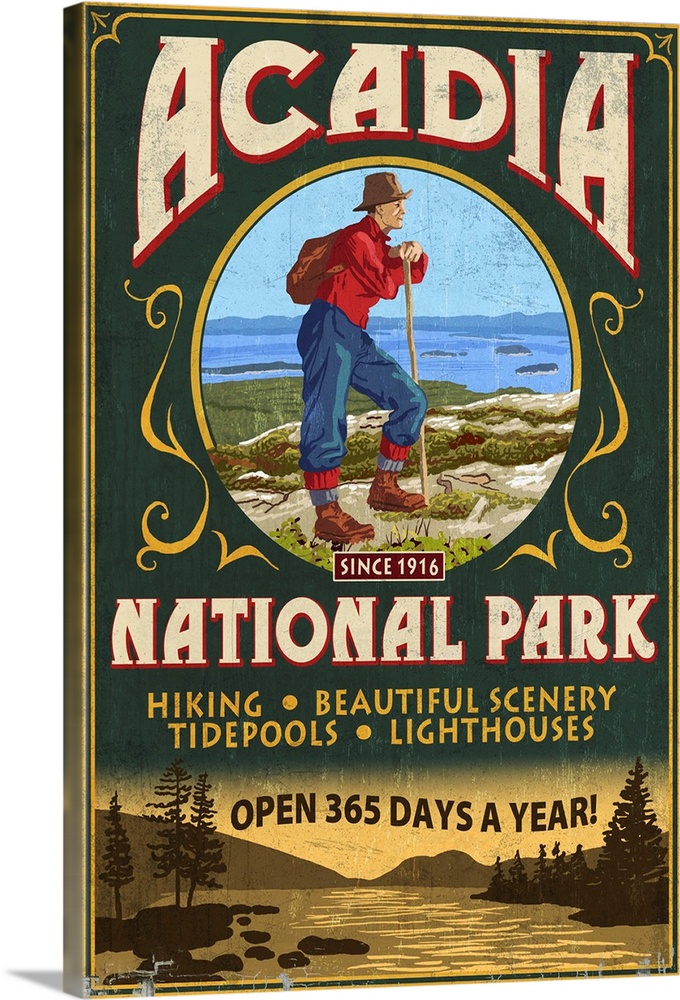This vintage-style poster for Acadia National Park features a prominently titled "Acadia" in white text with a red outline at the top, followed by "Since 1916 National Park" at the bottom. It is framed with a bright yellow border. In the center, the dark green background transitions seamlessly into a warm yellow, spotlighting the heart of the illustration where a round inset portrays a Caucasian hiker. The hiker, dressed in a red shirt and blue trousers with red and gray striped cuffs, and brown hiking boots, leans forward on his walking stick. He wears a brown backpack and a matching hat, standing against a backdrop of serene blue water. Complementing this central figure, the bottom section of the poster depicts a detailed yellow and brown silhouette of a tranquil forest scene, featuring trees, rocks, and a lake or river under a setting sun and yellow sky. Gold text here promotes the park's prime activities: hiking, beautiful scenery, tide pools, and lighthouses, emphasizing that Acadia National Park is open 365 days a year.